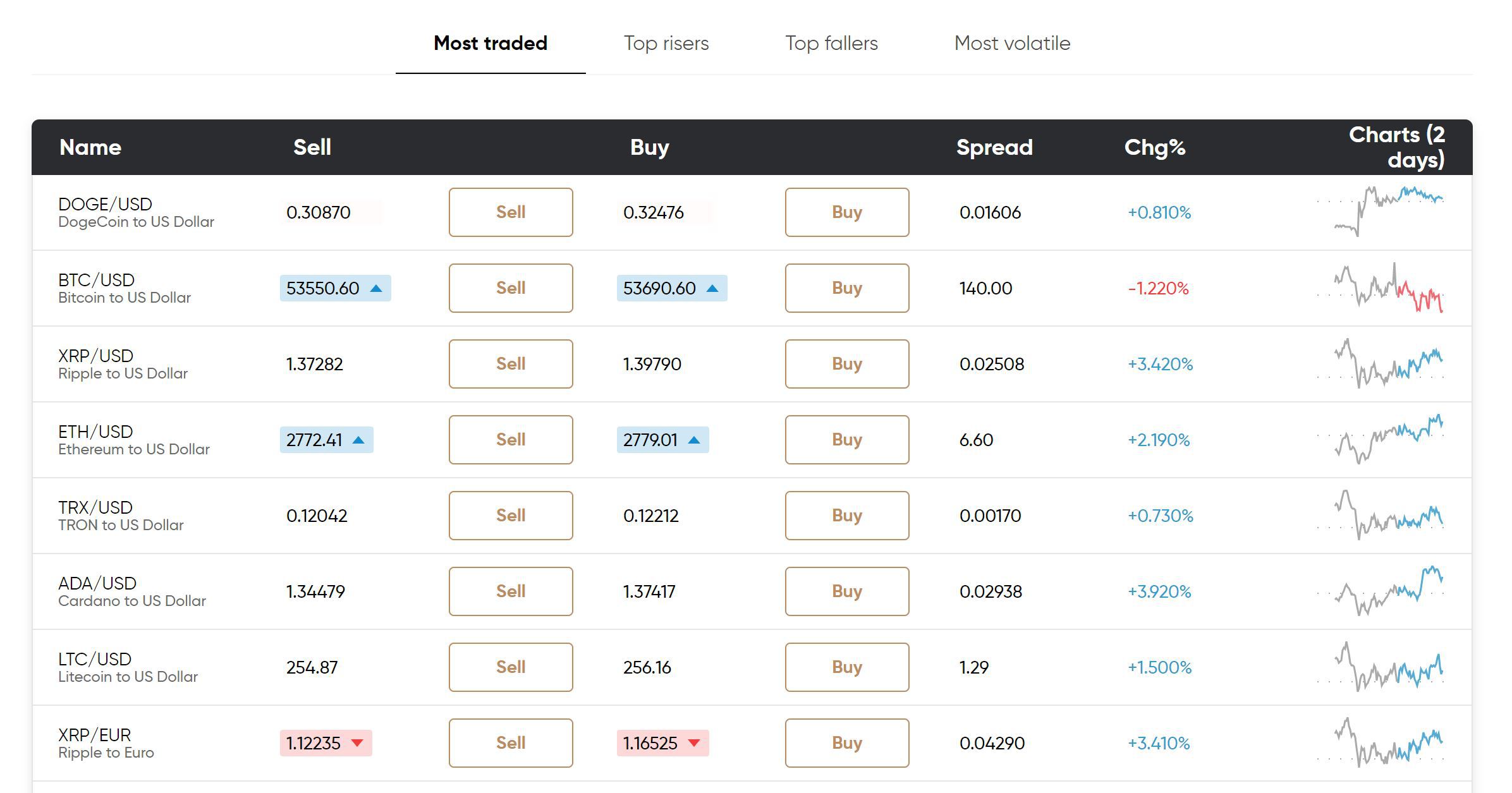This screenshot features a comprehensive cryptocurrency trading platform interface. The top section of the platform displays categorized lists: "Most Traded," "Top Risers," "Top Fallers," and "Most Volatile," with the "Most Traded" tab currently highlighted. 

Under the "Most Traded" category, the leading cryptocurrencies are prominently listed, starting with Dogecoin (DOGE) at the top, followed by Bitcoin (BTC), XRP (identified twice — suggesting possible repetition or an error), Ethereum (ETH), Tron (TRX), Cardano (ADA), and Litecoin (LTC).

Each cryptocurrency listed is accompanied by several key data columns including:
- **Sell Price:** The price at which the cryptocurrency can be sold.
- **Buy Price:** The price at which the cryptocurrency can be purchased.
- **Spread:** The difference between the sell and buy prices.
- **Percentage Change:** The fluctuation in price expressed as a percentage.
- **Price Trend Chart:** A small graphical representation illustrating the price trend over the past two days.

The platform's interface also allows users to directly execute buy or sell transactions through clearly marked options.

The overall design and features of this platform suggest it is user-friendly and likely popular among cryptocurrency traders, although the exact name of the application is not provided.